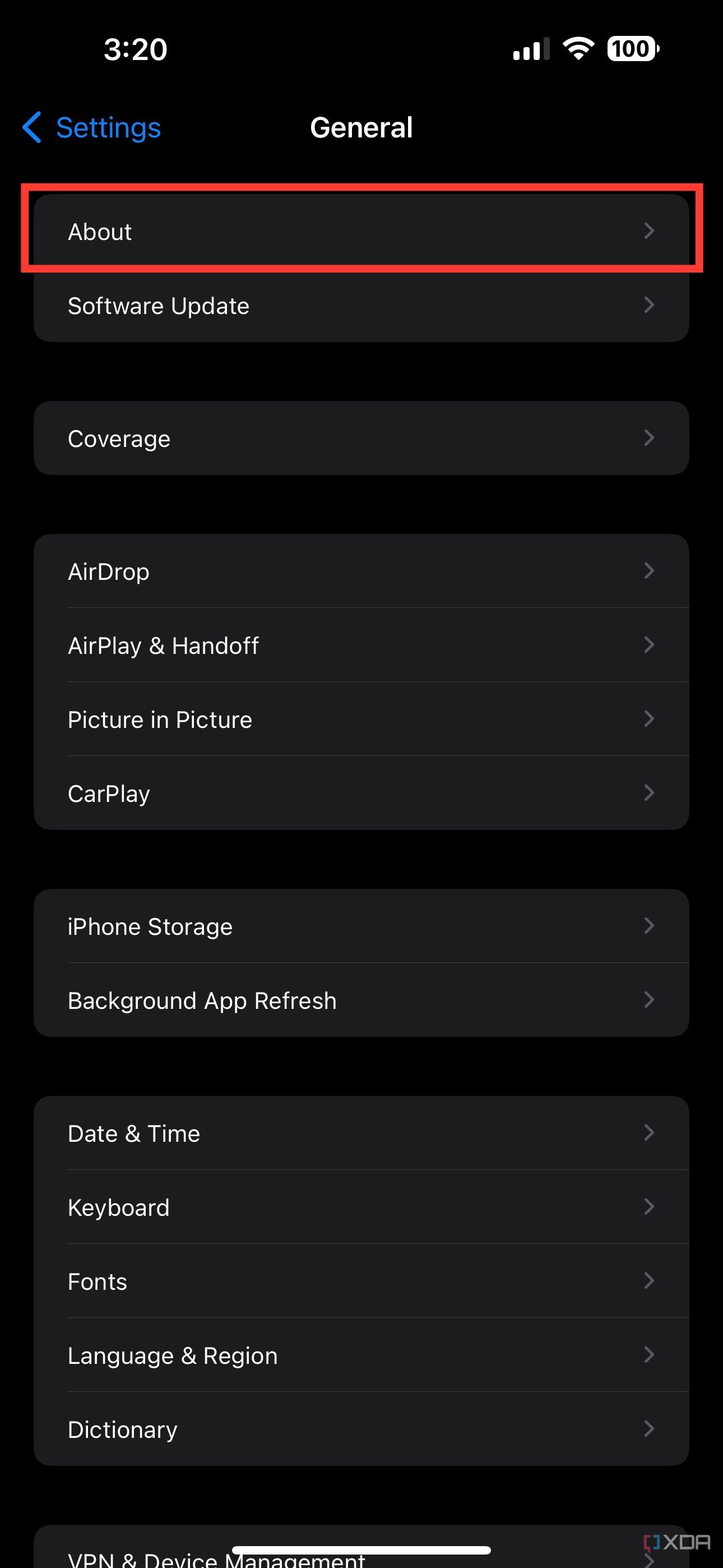The image features a black background with a smartphone screen showing a "Settings" menu. In the top left corner, the time is indicated as 3:20, and the status icons reveal a strong Wi-Fi signal and three out of four bars of reception, along with a fully charged battery at 100%. 

Beneath these icons, on the left-hand side, is a blue "Settings" label accompanied by a left-pointing arrow. The section below it is highlighted with a red outline and a gray background. 

This section includes the following options in white text:
- "About"
- "Software Update"
- "Coverage"
- "AirDrop"

Each item is separated by a thin gray line.

Subsequent menu items, each separated by thin gray lines, are listed as follows:
- "AirPlay & Handoff"
- "Picture in Picture"
- "CarPlay"
- "iPhone Storage"
- "Background App Refresh"
- "Date & Time"
- "Keyboard"
- "Fonts"
- "Language & Region"
- "Dictionary"

The detailed display of the settings menu indicates the phone's comprehensive user interface for managing various functionalities and preferences.